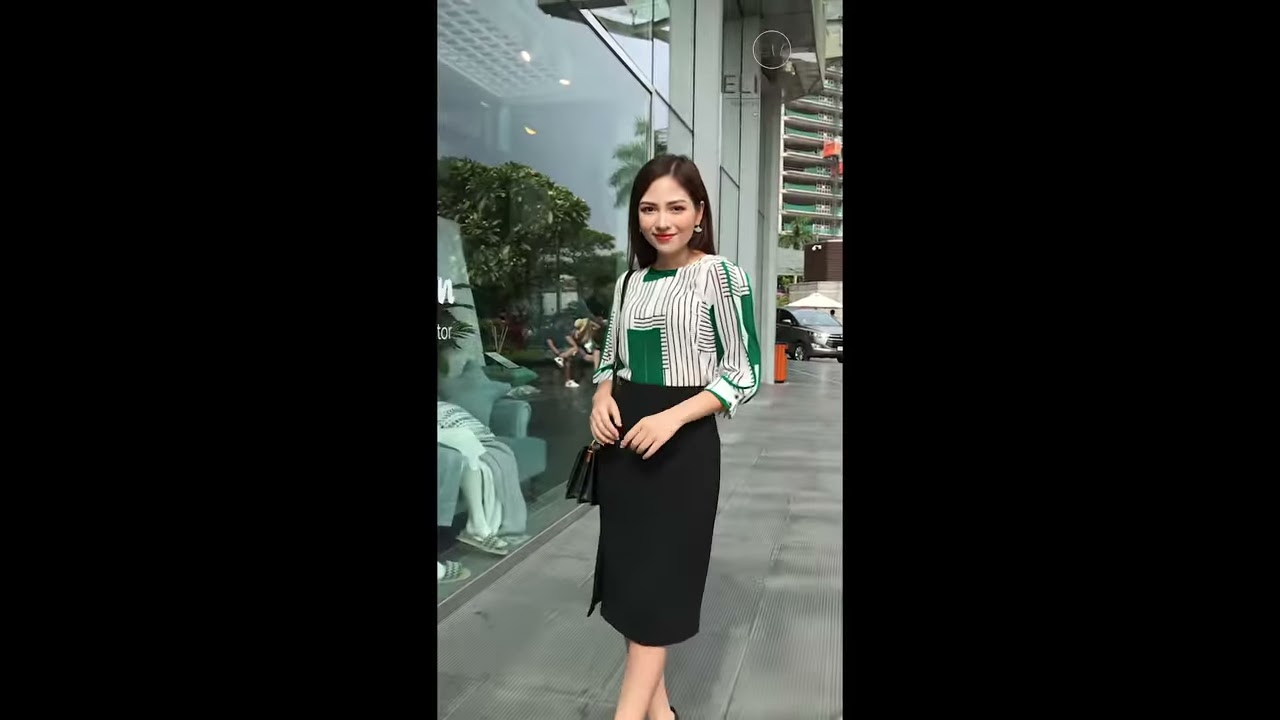A young Asian woman with straight, black, past-the-shoulder-length hair, stands on an empty sidewalk, posing confidently for the camera. She is wearing a fitted black pencil skirt that extends just below her knee and a white shirt adorned with horizontal stripes and green rectangular panels. Over her right shoulder, she carries a black handbag with a matching strap. Her hands are clasped in front of her, with her left leg slightly overlapping her right, emphasizing her relaxed yet intentional pose. She smiles warmly, her lips painted with lipstick, and a single earring catches the light. The woman is positioned in front of a large glass storefront window, which displays a chair. To her right, further down the sunny and dry sidewalk, are visible elements of an urban cityscape: a dark-colored car, an orange trash can, a tree, and a multi-level commercial building. The scene is framed by thick black lines on either side, focusing the attention on her as she stands against the backdrop of city life.